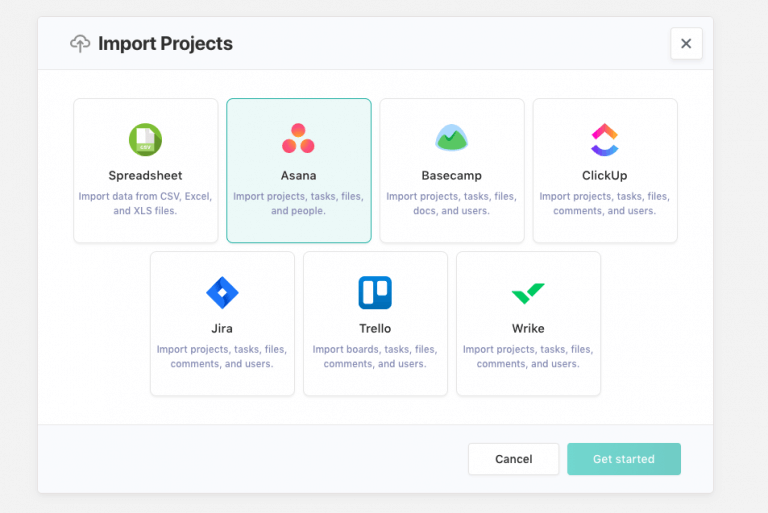In this image, we are presented with a screenshot. The screenshot is a horizontally extended rectangle set against a solid light gray background. Displayed on the screen is an open white page. At the top left corner of the page, the header reads "Import Projects" in bold black text. To the left of the header is an icon depicting a cloud with an upward arrow.

Below the header, within a distinct white background area, there are four horizontally aligned boxes. The first box is white inside and contains text indicating "Spreadsheet Import: data from CSV, Excel, and XLS files." The second box, which is highlighted and outlined in blue, reads "Asana" with three vertical red dots beside the text. The third box features an icon of a green mountain against a blue sky, with the text "Basecamp." The fourth and final box in this row is labeled "ClickUp."

Beneath these four boxes are three additional squares arranged horizontally. The first square reads "JIRA," the second says "Trello," and the third is labeled "Wrike." These options are accompanied by the text, "Import projects, tasks, files, comments, and users," which suggests the functionalities available for the listed platforms and tools.